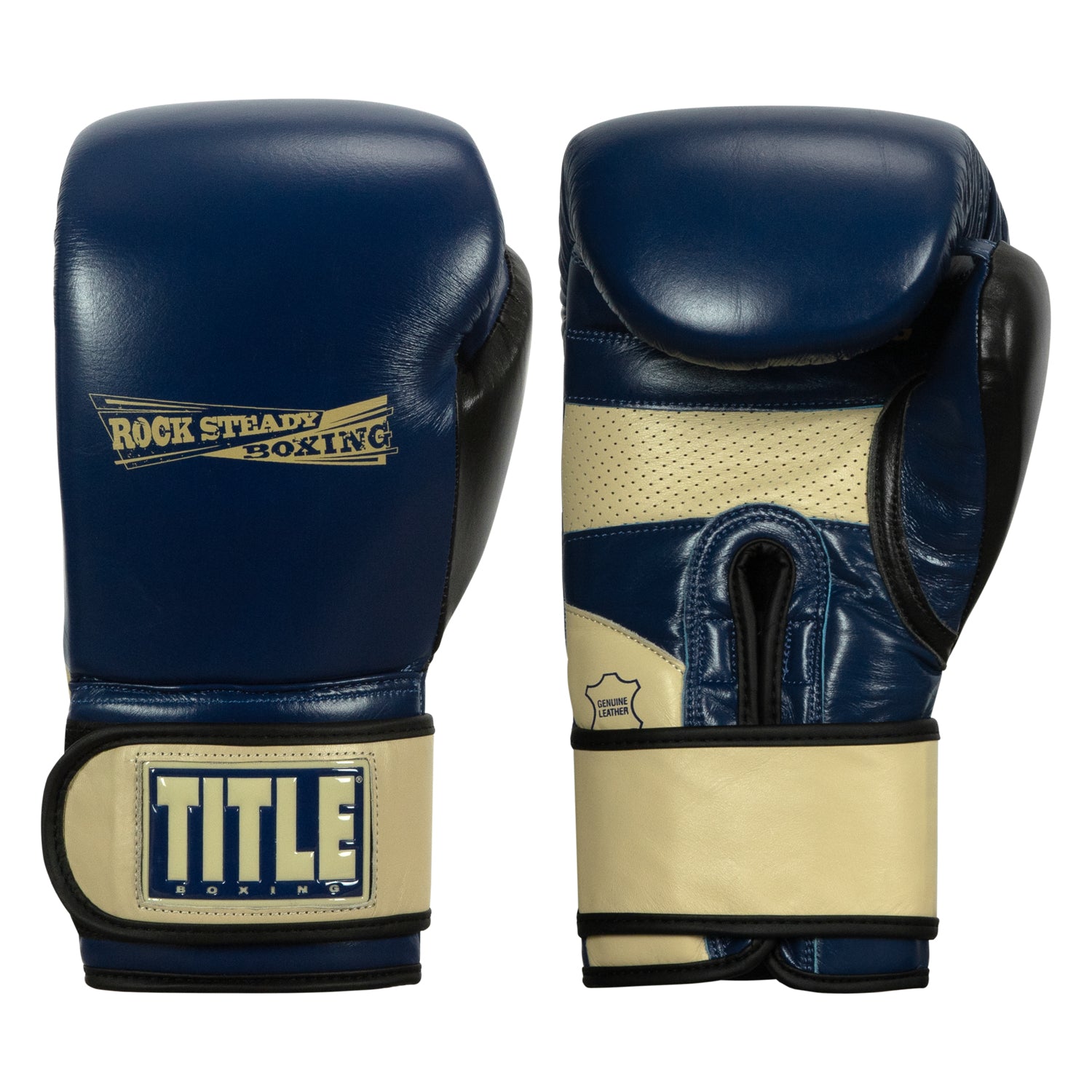The image depicts a product photo of a pair of blue boxing gloves, meticulously isolated against a featureless white background, creating the illusion that the gloves are floating. The pair consists of a left-hand glove, presented with its back visible, and a right-hand glove, displaying its palm side. Both gloves are identical except for their mirrored orientation.

The gloves prominently feature "Rock Steady Boxing" in tan lettering on their backs. The left glove's palm remains unseen, highlighting the padded, durable upper side designed to cover the top of the hand and wrist. The right glove reveals the intricately segmented palm area, constructed to facilitate comfort and ventilation. This area includes a yellow leather bar with small black ventilation holes, presumably to allow airflow and wick away sweat.

For wrist support, each glove is equipped with an adjustable strap, tan with black borders. This strap secures the gloves snugly to the wrists using a Velcro closure. On the strap, located at the back of the wrist, is a prominent rectangular patch with a blue background adorned with the glaring white text, "Title Boxing."

Additional details include a yellow leather triangle with "BOXING" written in black text centrally positioned on the back of each glove, and a small U-shaped opening on the palm side of the right glove to facilitate the insertion of the hand. The thumb compartments are designed to hold the thumb close to the fingers, ensuring both security and ease of movement.

Overall, these gloves are polished to combine aesthetics with functionality, with detailed features that cater to both comfort and durability during rigorous boxing sessions.